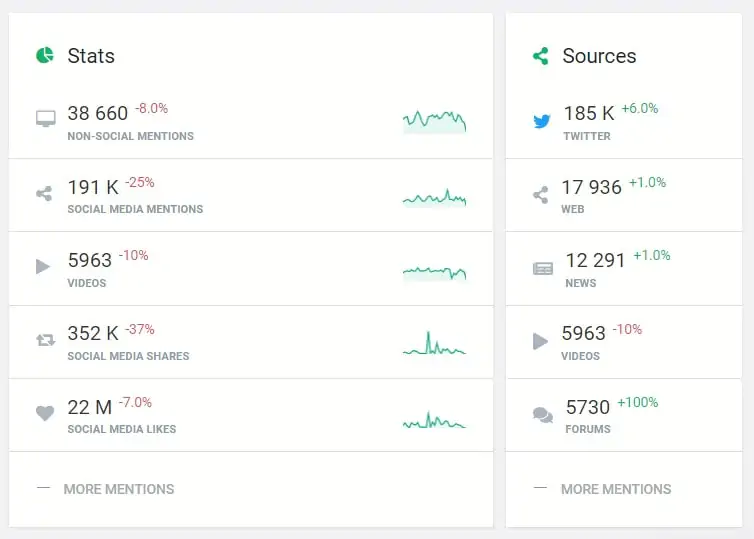A detailed view of a pop-up screen showcases comprehensive social media statistics and their sources. On the left, under the heading "Stats," the following metrics are displayed in descending order: 38,669 social mentions, 191k social media mentions, 5,963 videos, 352k social media shares, and 22 million social media likes, followed by a note for "more mentions". On the right, under "Sources," the data indicates contributions from various platforms: 185k from Twitter, 17,936 from web sources, 12,291 from news outlets, 5,963 from videos, and 5,730 from forums, also followed by "more mentions". The left-side metrics are shown in red, indicating a decline in these figures, while the right-side metrics are highlighted in green, demonstrating a positive increase.